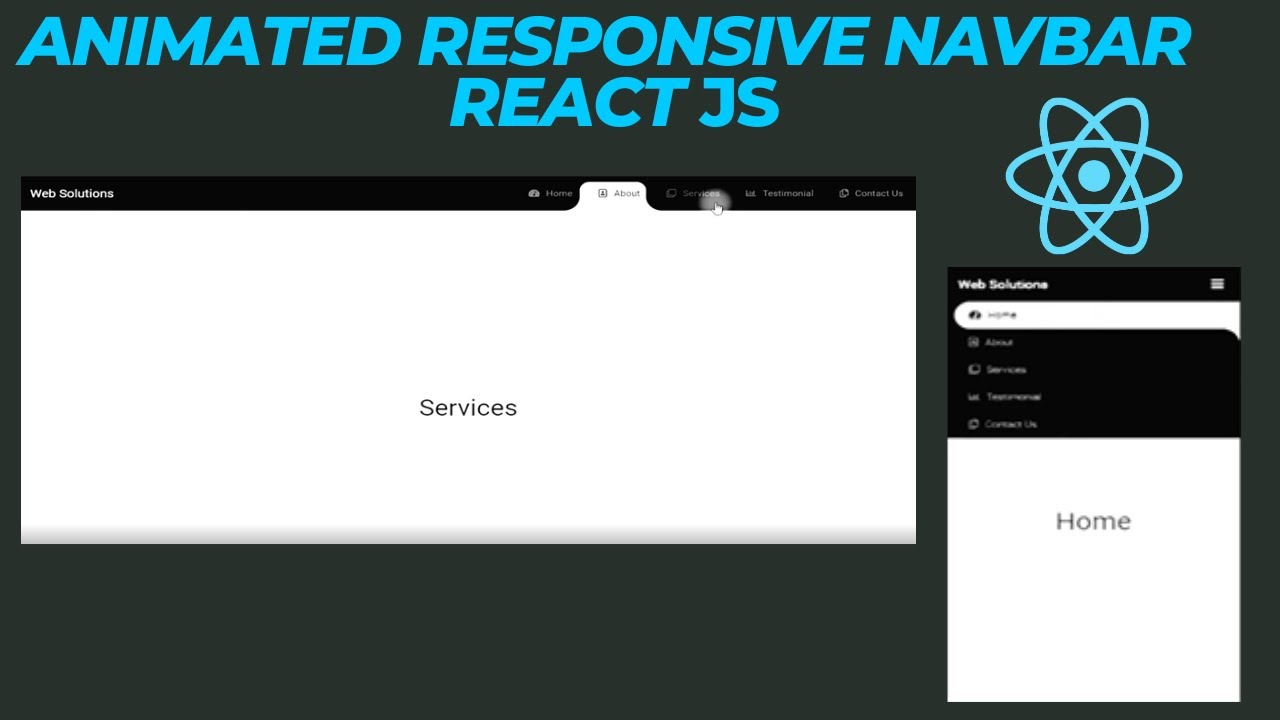**Caption:**

The image features a user interface with a dark gray background. At the top, in Carolina blue, bold, uppercase letters, it reads "ANIMATED RESPONSIVE NAVBAR REACT JS." To the right of this text, there is a light blue icon resembling an atom, characterized by a central circle with three overlapping ovals horizontally and diagonally. On the left, set against a black background, the text "Web Solution" is displayed. 

There is a tab labeled "About" situated at the top on a white background, and centered in black letters is the word "Services." Below the atom icon, "Web Solutions" is written, followed by five entries that are too blurry to discern, except for the top one which stands out with a white border, unlike the rest which are black. Below this section is a large white square containing the word "Home" written in gray text at the center.